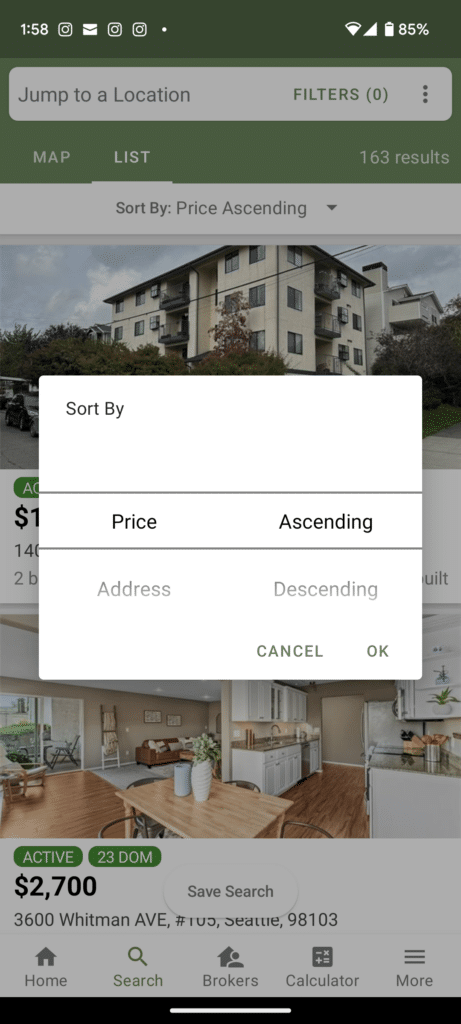This is a detailed screenshot of a smartphone displaying a real estate website. The phone's status bar features a dark green top inch, with a white "158" on the left side, followed by a camera icon, an email icon, two additional camera icons, and a white dot. On the right side of the status bar, it shows "85%" battery life, with battery, internet, and Wi-Fi icons all indicating full connectivity.

Just below the status bar, there's a lighter green section about an inch and a half in height. At the top of this section, there is a gray search bar containing the text "Jump to location" in black font. To the right of the search bar, the word "Filters" is displayed with a "(0)" next to it and a vertical ellipsis (three dots) for additional options.

Beneath the search bar, the interface changes to white, displaying tabs labeled "Map" and "List". On the right side of these tabs, it shows "163 results". Underneath this white border, there’s an option for "Sort by price ascending".

There is then a large area showing a real estate listing. The top image depicts a brown building against a cloudy sky with a bit of grass in the foreground. This image is partially overlaid by a white pop-up square that obscures its bottom half. Below this picture, you can see the edge of another image through the overlay. This partially visible image features an interior scene with hardwood floors, brown tables, and white flower pots, along with some kitchen utensils.

The content within the white pop-up is as follows: the top left corner reads "Sort by" in black text. A gray line runs horizontally below this, followed by options "Price" on the left and "Ascending" on the right in black font. Another gray line below these options separates the next set of options, which indicate "Address" on the left and "Descending" on the right. Below "Descending", there are two clickable options labeled "Cancel" and "Okay".

Beneath this pop-up, there is additional information about the cost and address of the listed properties, partially visible in the screenshot.